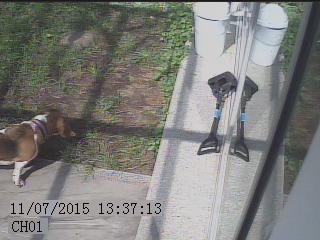The image, captured by a security camera on the side of a residence, shows a driveway with a patch of grass next to it. On the left-hand side, a white and brown beagle dog is standing, wearing a collar and looking towards a white cylindrical structure. This structure features two barrel-shaped components and appears elevated, revealing grass underneath. Above the cylindrical structure, black objects with handles, resembling shovels, can be seen. To the right side of the image, near what appears to be a window or sliding door, there is a white bucket. The bottom left corner of the image displays a timestamp: 11-07-2015, 13:37:13, with "CH01" written underneath it. The natural sunlight enhances the visibility and detail of this outdoor scene.